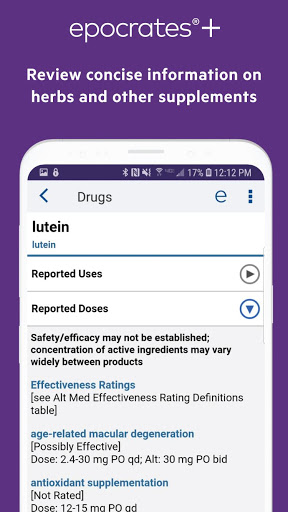This image is a detailed screenshot of an advertisement for a mobile application named Epocrates+. The background of the ad is predominantly purple with text in white, making the content stand out effectively. At the very top of the advertisement, "Epocrates+" is prominently displayed, indicating the name of the application.

Central to the advertisement is a large image of a smartphone, showcasing the app's interface. The screen of the phone is focused on the section for drugs and supplements, highlighting its utility for medical professionals or individuals interested in detailed drug information. 

Under the app's name, there is a tagline that reads, “Review concise information on herbs and other supplements,” indicating that the application provides succinct and essential details about various herbal products and supplements.

The phone display shows an entry for "Lutein," detailing its uses and efficacy. Specifically, the screen includes sections such as "Reported Uses," "Reported Doses," and warnings that "Safety and efficacy may not be established," and that "Concentration of active ingredients may vary widely between products." Additionally, it provides "Effectiveness Ratings" for conditions such as age-related macular degeneration and antioxidant supplementation.

Overall, the advertisement effectively conveys that Epocrates+ is a comprehensive resource for drug and supplement information, depicted through a visually appealing and informative presentation.